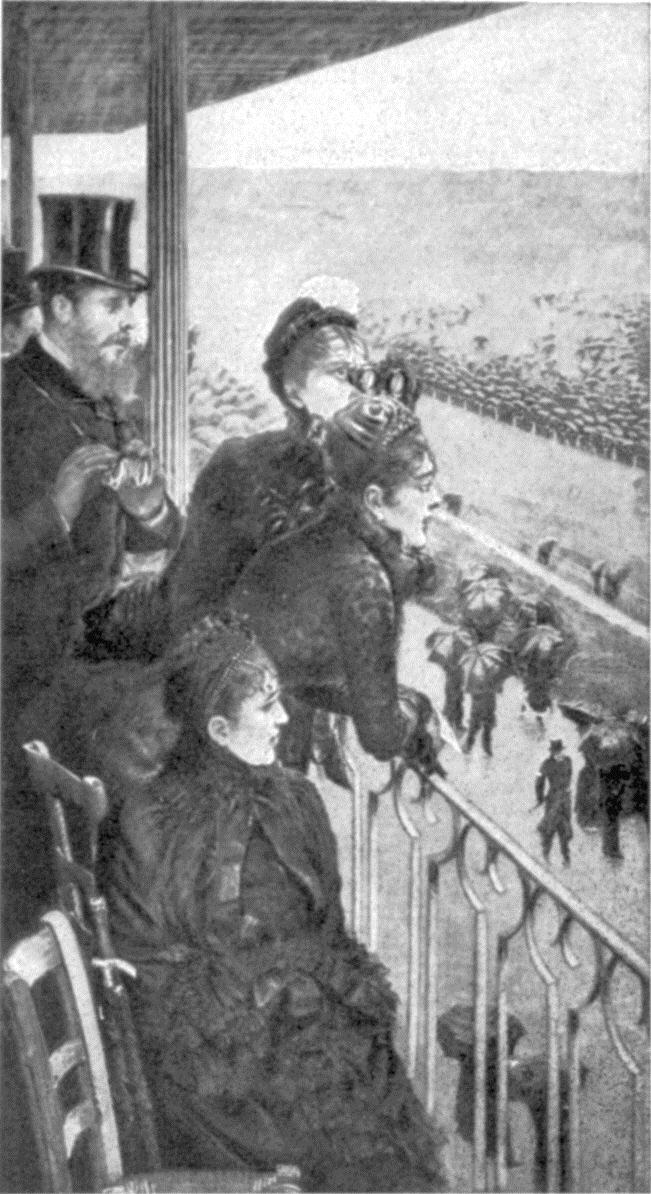This monochrome painting, likely a reproduction of a 19th-century scene, features a detailed depiction of a racecourse setting viewed from an elevated balcony. The composition includes three elegantly dressed women and a distinguished man, all attired in period clothing. The man, positioned at the rear, sports a top hat, a beard, and a mustache, and wears what appears to be a formal suit. He holds binoculars close to his chest. 

In the foreground, a woman dressed in a long, dark dress adorned with feathers is seated, with an empty chair beside her. Her companions, two other women, are adorned in similar 19th-century attire and hats, and they lean against the balcony railing. One of these women is seen peering through binoculars, presumably observing the racetrack below. 

The racecourse itself is visible in the distance, though no horses are present. Spectators line the edge of the track, and directly below the balcony, several individuals stroll along, many carrying umbrellas. All of this unfolds under a somber, gray sky, enhancing the monochrome aesthetic of the artwork.